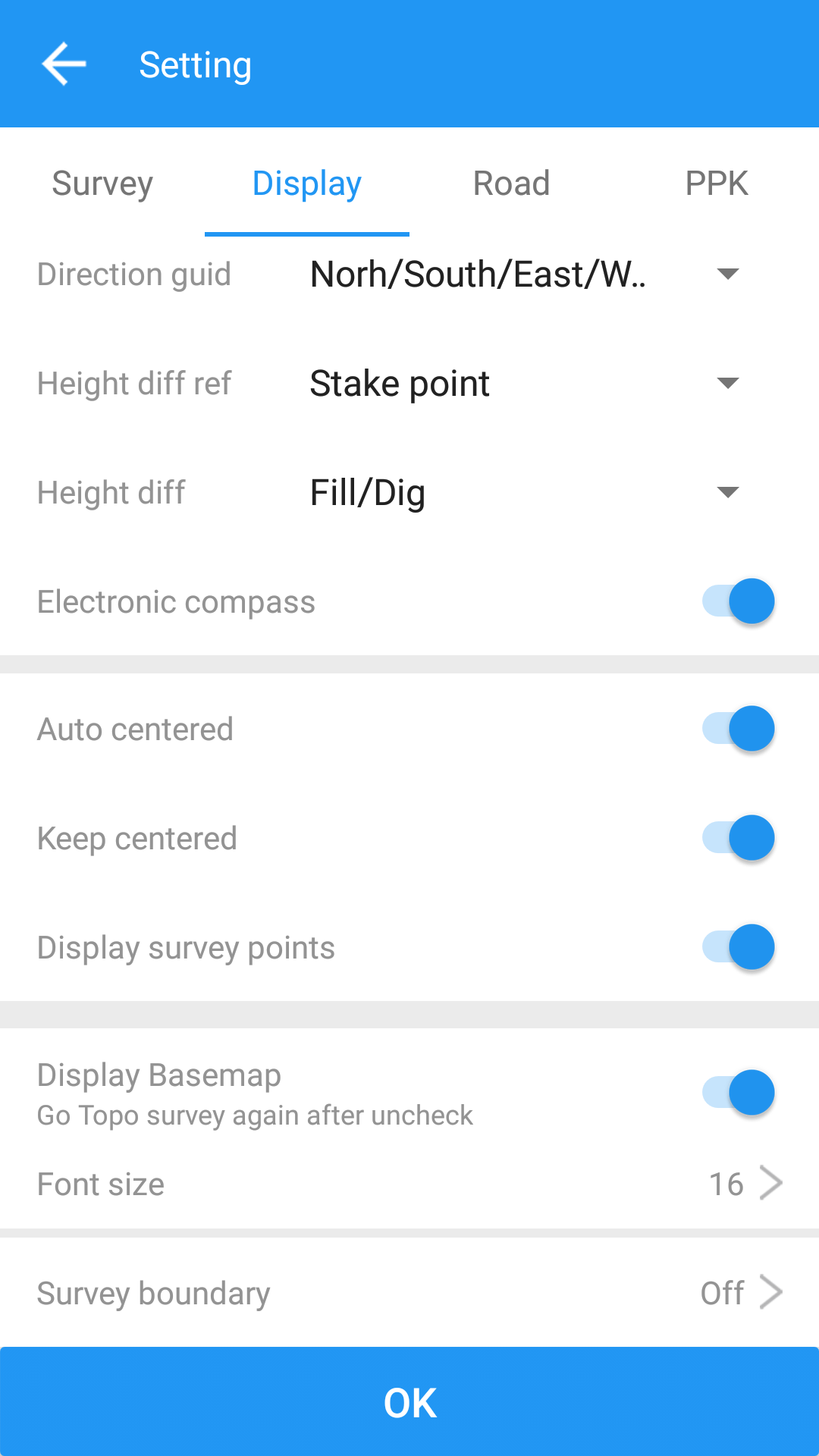This screenshot from an unidentified mobile device, whether Android or iPhone, showcases the settings section of an unidentified application. The interface features a minimalist design with a predominantly white and light grey background. Grey text is used for descriptive labels and instructions, while actionable items are highlighted in blue.

At the top of the screen, a blue banner with the white text "SETTING" includes a left-pointing arrow, indicating a navigation option. Directly underneath, four horizontally arranged tabs offer different configuration categories. These tabs are labeled "Survey," "Display," "Road," and "PPK." The selected tab, "Display," is emphasized with blue text and a corresponding underline.

The contents of the "Display" tab are organized as follows:

1. **Direction Guide:** Options listed are "North/South/East/West."
2. **Height Differential Reference:** The selected reference is "Stake Point."

Below these sections, several options are presented with toggles for enabling or disabling features. These toggles appear blue, indicating they are activated:
- **Auto-Centered**
- **Keep Centered**
- **Display Survey Points**

Each of these toggle options has been turned on, as evidenced by their blue color.

At the bottom of the screen, a large blue rectangular button stretches across the width, bearing the white text "OK," which likely serves to confirm any changes made within this settings section.